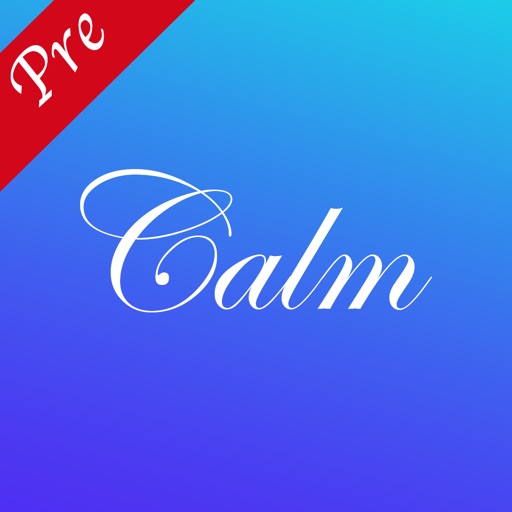The image features a large blue square with a gradient background transitioning from a light Tiffany blue at the top to a deep royal blue at the bottom. Dominating the center of this gradient background is the word "CALM" in a highly stylized, cursive script. The letters are white and italicized, leaning gently to the right, with the capital "C" being particularly elaborate, adorned with intricate curls and flourishes.

Located in the upper left-hand corner of the image, a diagonal red ribbon or band slices across the blue, creating a triangular blue segment at the very top corner. This red band extends about a third of the way down the left side and a third of the way across the top of the square. Inside the band, written in matching cursive white script, is the word "PRE," situated at a 45-degree angle in alignment with the band.

The overall composition, though somewhat minimalistic, emphasizes the boldness of the word "CALM" and the striking contrast created by the red ribbon against the varying shades of blue.